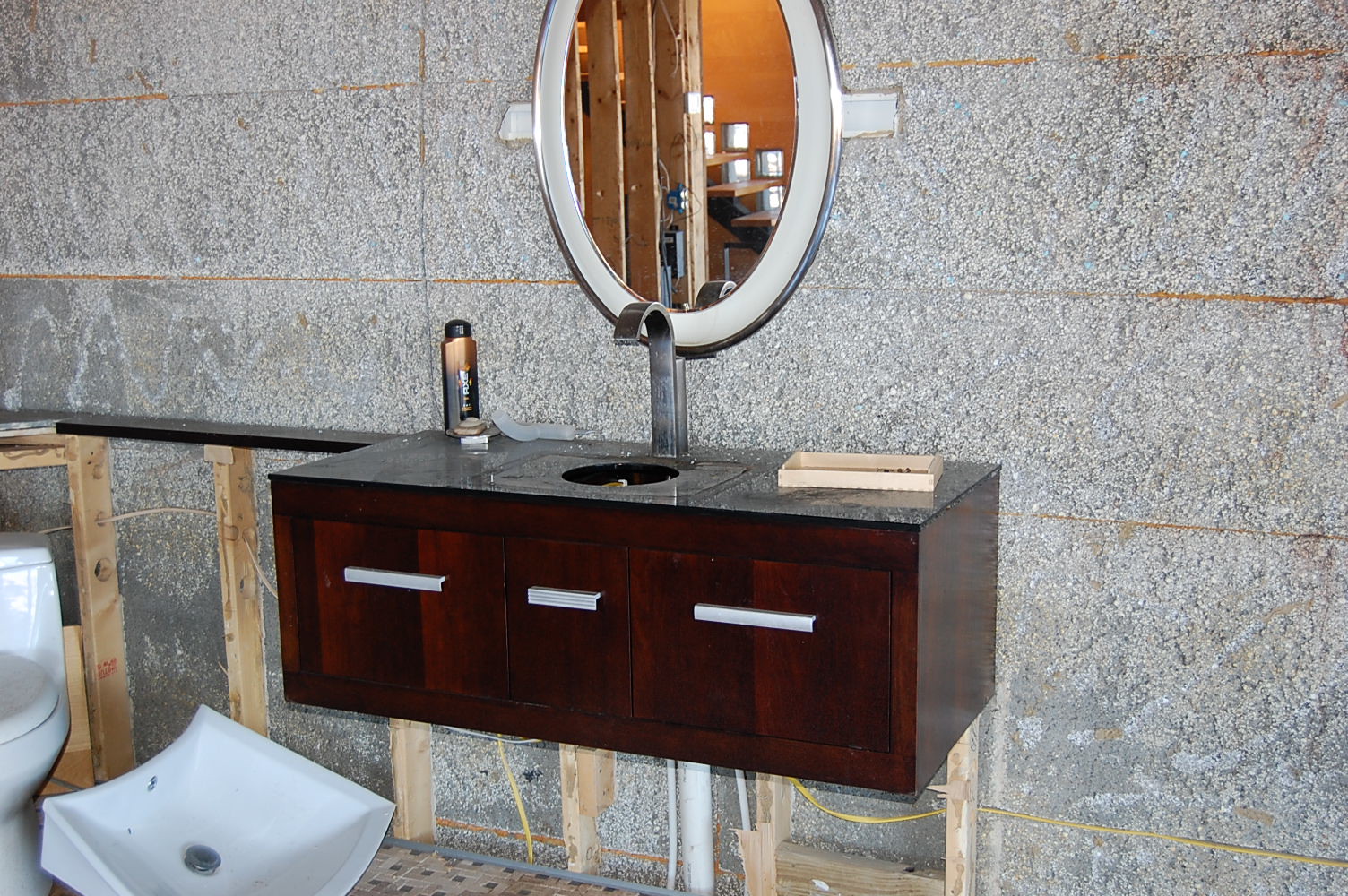This image showcases a bathroom under construction. A striking tile wall, possibly made of quartz or marble, serves as the backdrop. The grout between the tiles has a distinctive orange hue. Centrally positioned is a contemporary floating vanity made of dark wood, featuring three sleek silver handles on its front. Above the vanity hangs an illuminated oval mirror, partially obscured at the top, reflecting wooden beams and several cans of paint. The faucet on the vanity rises and curves into a U-shape, but notably, the sink that should be on the vanity is instead on the floor. This sink is an unusual square shape with two angled sides and a curved edge. To the left of the vanity, wooden beams support a wooden shelf, and part of a white toilet is visible in the scene.